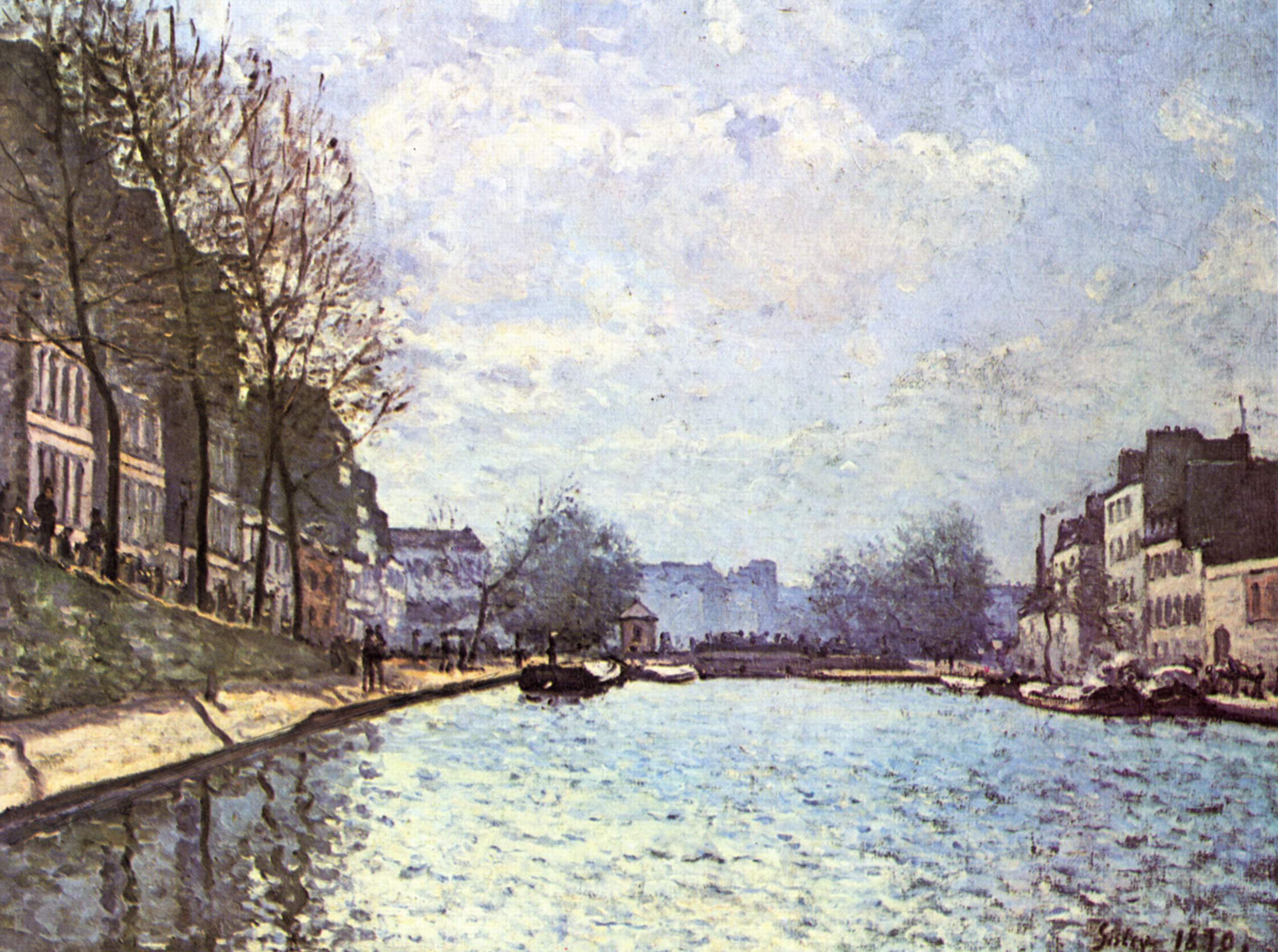The image portrays an impressionistic scene reminiscent of a Monet painting, capturing a river flanked by continental European-style buildings which evoke a sense of being in France or perhaps the Netherlands. The painting features a waterway with barges moored along the edges, tied by a cement path, particularly prominent on the left side. Surrounding the river is a serene setting with tall, ornate buildings on the left and shorter, multi-story old buildings on the right. The left side also includes a flat walkway leading to a gentle incline covered by tall trees, contributing to the scenic beauty. People are visible near the buildings and along the walkway, adding life to the scene. The sky above is a muted blue, dotted with soft, fluffy clouds, complementing the vibrant blue of the water which sparkles under the sunlight. The painting’s colors include blue, white, gray, and some green, creating a harmonious palette. At the bottom right corner of the artwork is a signature that appears to read "Sister," with the year 1850 inscribed next to it.